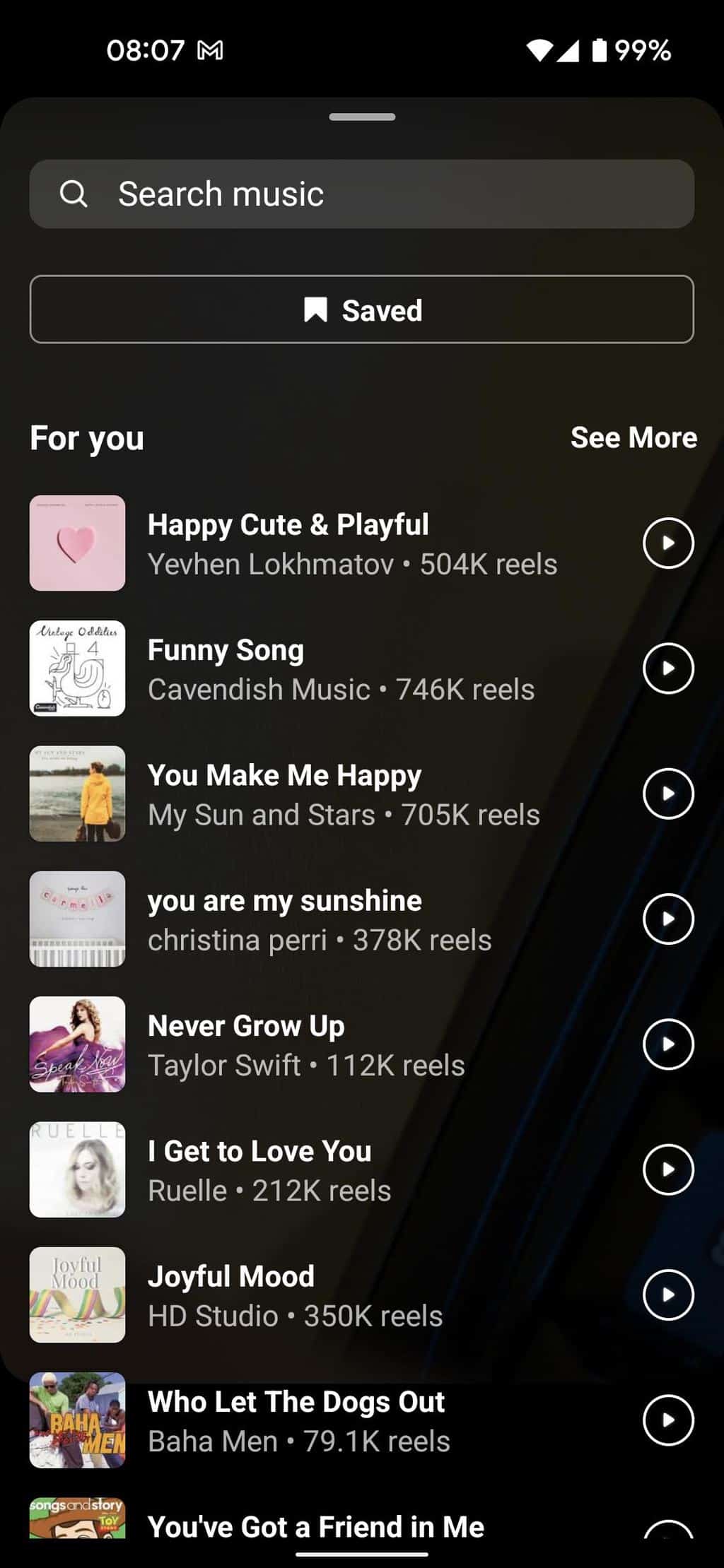This image is a screenshot of a music list taken on a cell phone, specifically showing search results for music recommendations. At the top left corner, it features the label "For You" with associated music icons. In the top right corner, there's a "See More" option available for further exploration. The list highlights categories like "Happy," "Cute," and "Playful," each represented by a square icon with a heart symbol inside it. The displayed tracks include notable titles such as "You Make Me So Happy," "I Get to Love You," "Never Grow Up" by Taylor Swift, "A Thousand Years" by Christina Perri, "You Are My Sunshine," "Joyful Mood" by HG Studio, "Who Let the Dogs Out" by Baha Men, and "You've Got a Friend in Me." The text is primarily in white against a black background, with lighter white text below the main list items. Each song entry also features a white circle with a white arrow inside it for action options. Additionally, the phone's status details are visible, showing a 99% battery level and a time stamp of 8:07. There are ten songs listed in total.